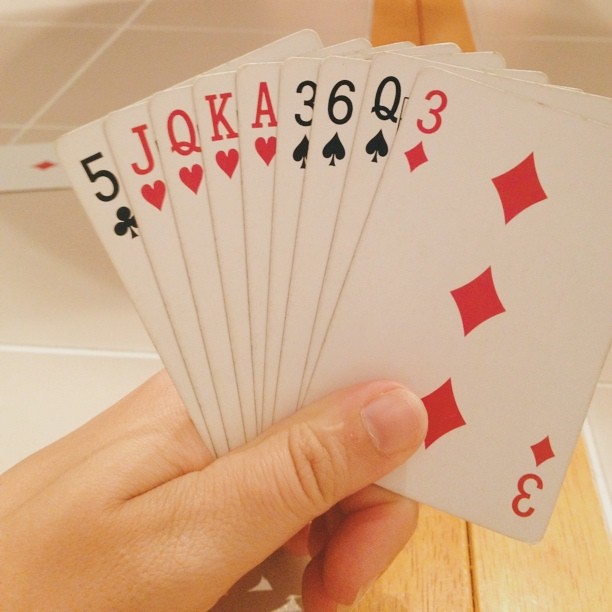In the image, a person's left hand, identifiable as belonging to a white individual, is holding nine playing cards. The cards are arranged from left to right as follows: a five of clubs (black), a jack of hearts (red), a queen of hearts (red), a king of hearts (red), an ace of hearts (red), a three of spades (black), a six of spades (black), a queen of spades (black), and a three of diamonds (red). On the table in the background, there is an ace of diamonds, identifiable by its single diamond symbol, though the ace mark is not visible. The table itself is distinct, featuring a surface of white tiles bordered by brown wood. The scene suggests the individual is engaged in a game of cards, possibly spades or poker.